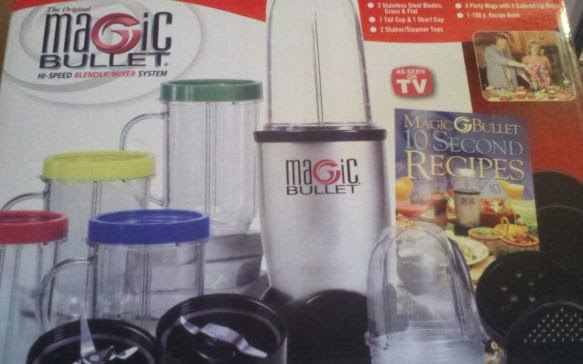The image showcases several Magic Bullet products prominently displayed, suggesting a promotional setup, possibly for a TV infomercial or trade show. At the center of the image is the Magic Bullet blender with a cap on, identifiable by its silver base and blending top. The branding is notable, with the word "Magic Bullet" displayed, featuring a red, enlarged "G". To the left of the blender, there are several clear cups with handles, each topped with differently colored caps: red, yellow, blue, and green. In the bottom left, the blender's chopper blades are visible, indicating the appliance is open. In the background, a product package reads "Magic Bullet High Speed Blender Mixer System", reinforcing the promotional theme. To the right side, a cookbook titled "Magic Bullet 10 Second Recipes", with images of various foods and drinks, is displayed, enhancing the product's appeal. The general setting appears indoors, with a slightly grainy quality, consistent with early 2000s promotional materials.